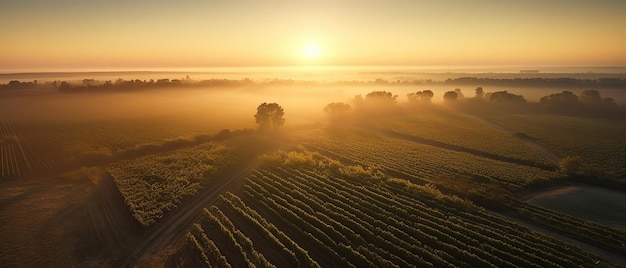This aerial photograph captures an expansive view of farmland blanketed in thick fog, likely taken during the early morning or evening hours. The green, leafy crops are meticulously arranged in vertical rows, with some diagonal sections visible, stretching across the land and leading up to a river at the edge. A prominent dirt path cuts through the crops, flanked by several trees. The horizon features a bright yellow sun, positioned in the middle of the image, casting a golden hue over the fog-laden landscape and turning the entire sky and river below a warm yellow. The mist creates a surreal atmosphere, enveloping distant buildings and blurring them into the fog. This ethereal scene is accentuated by a series of white lines formed by the sun's rays piercing through the dense fog, illuminating the farmland and adding depth to the serene, almost dreamlike setting.